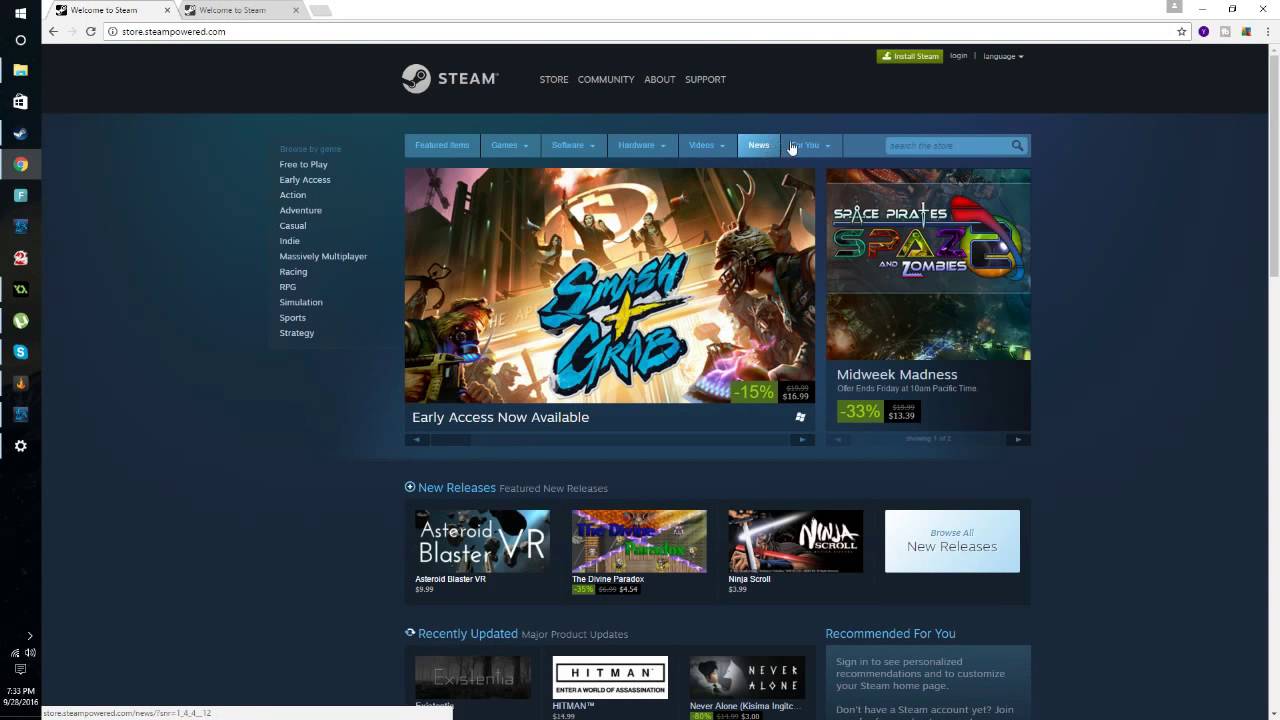The image depicts a computer screen with three browser tabs open, two of which clearly display the "Welcome STEAM" page. The third tab is not visible in detail. The currently active tab features the STEAM homepage, which is not fully loaded, as indicated by the prominent olive green button at the top with the prompt to "Click to Install STEAM." The web address visible in the search bar is "store.steampowered.com."

At the top navigation of the page, several menu options are displayed: "STORE," "COMMUNITY," "ABOUT," and "SUPPORT." An advertisement banner showcases "Early Access Now Available," featuring a picture of "Smash and Grab." To the right of this, other games such as "Spice Pirates and Zombies" and a "Midweek Madness" promotion are highlighted.

Further down the page, the "New Releases" section is prominently featured with titles like "Asteroid Blaster VR," "The Divine Paradox," and "Ninja Scroll," along with an option to browse all new releases. Below this section, there's a list of recently updated games. On the left side of the screen, there is a vertical navigation column offering additional browsing options.